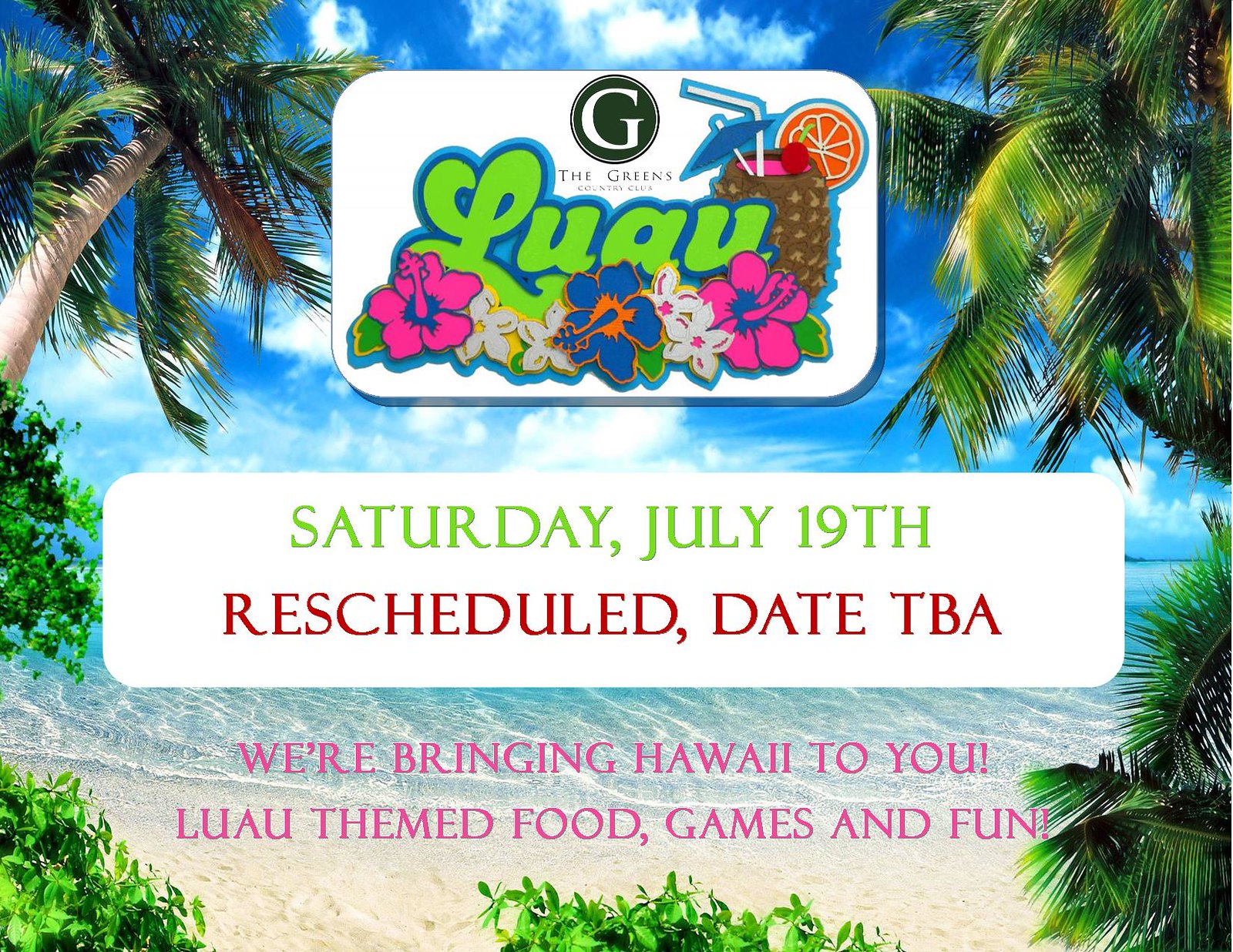This vibrant advertisement invites you to the Greens Country Club Luau, set against a stunning tropical backdrop that spans the entire image. The scenery showcases a lush paradise with palm trees on either side, a radiant blue sky dotted with white clouds, and a gradient stretch of water from clear to deep blue leading down to a nearly white sandy beach. At the top center, the headline reads "The Greens Country Club Luau," adorned with tropical flowers and a pineapple cup filled with a pink drink, complete with a straw and umbrella. Below, a white lozenge-shaped banner displays the event's original date, "Saturday, July 19," followed by "rescheduled, date TBA." Further down, in vivid pink letters, the text promises, "We're bringing Hawaii to you: luau-themed food, games, and fun." The ad is rich with colors including green, blue, pink, orange, and red, accentuated by earthy tones in the trees and drink, capturing the essence of a Hawaiian escapade. An inset on the lower left announces "The Greens Luau," embellished with hibiscus flowers and a tropical drink, tying the theme together with promises of an unforgettable event.